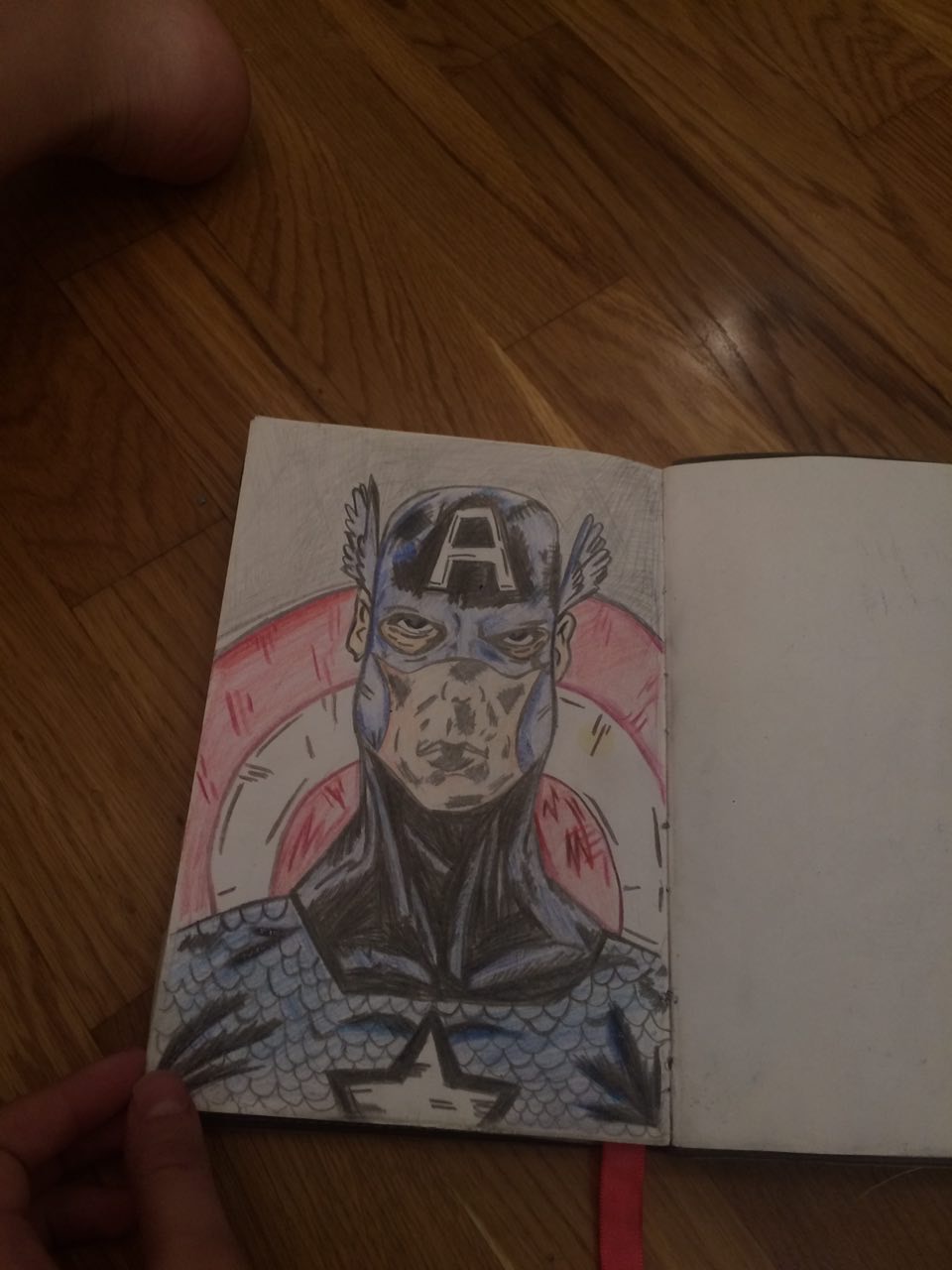The photograph depicts an indoor setting with a wooden floor that features prominent wood grain patterns. A person is sitting on the floor, and their heel is visible in the upper left corner of the image. In the lower left corner, the person's thumb and index finger are seen holding a page of a small, blank sketchbook open. The right-hand page of the sketchbook contains a detailed, colored pencil illustration of Captain America. The superhero is depicted in his classic attire, including a blue bodysuit, a blue mask, a white star on his chest, and an 'A' on his forehead. Additional details such as white wings on either side of his helmet and a skin-toned face are present. Behind Captain America, a red and white bullseye pattern, representing his iconic shield, provides a striking backdrop against the wooden surface. The image is predominantly dark, contributing to the overall mood and emphasizing the details of the sketch and the texture of the wooden floor.